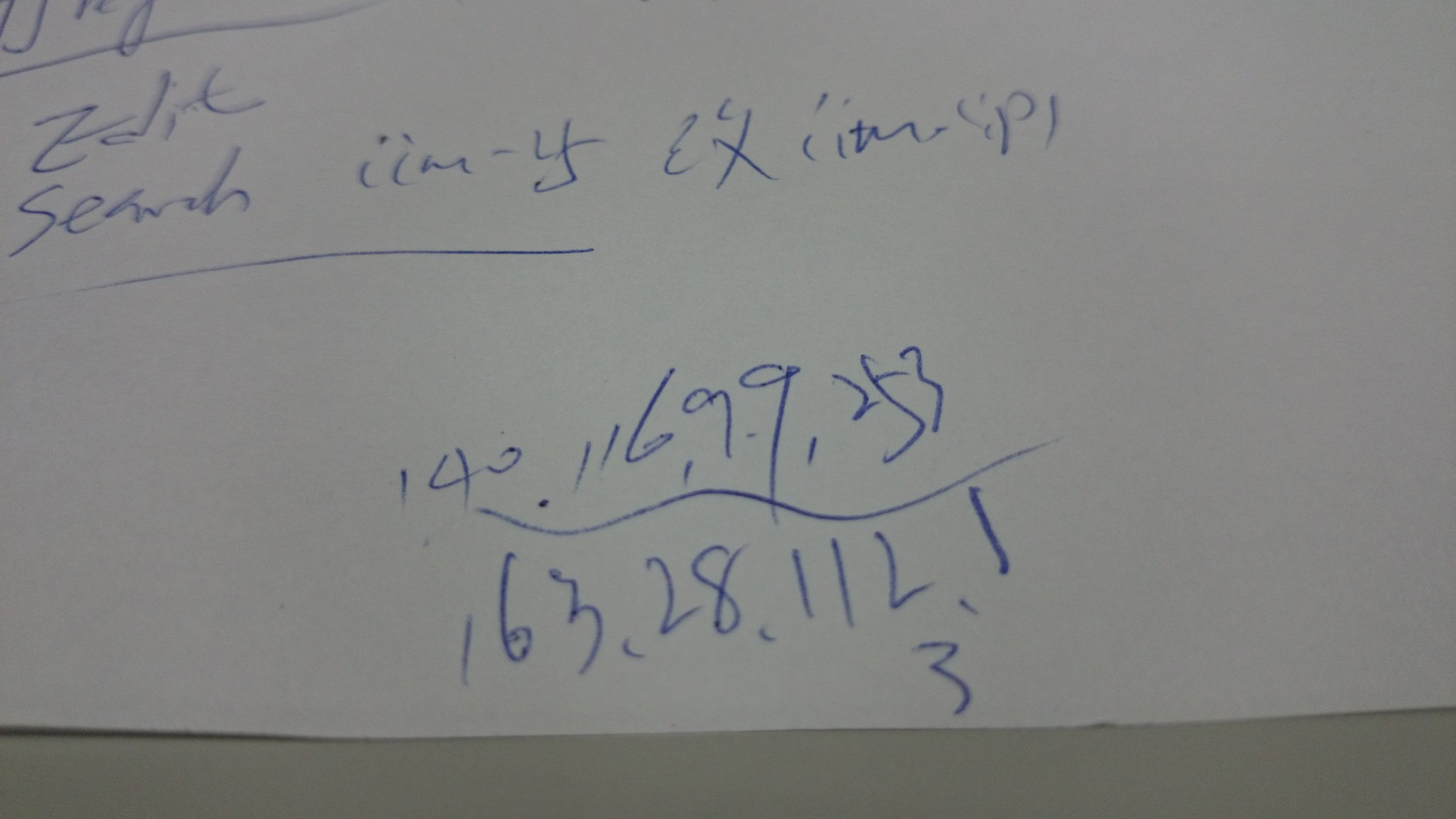In a dimly lit setting, this close-up photograph captures a small section of a white sheet of thin, standard printing paper with a rectangular shape. The paper rests on a light gray surface, and its bottom left and right corners appear slightly wrinkled or curled. A small notch is visible along the bottom edge. The paper features multiple lines of handwritten blue ink. The readable text includes: "edit, search. I, I, M, minus Y, I, X, I, I, M, I, P." Below this, there is a sequence of numbers: "140.116, 99, 253," underlined with a squiggled blue line. Beneath this underlined section are additional numbers: "163, 28, 112, 13." The rest of the paper remains blank.